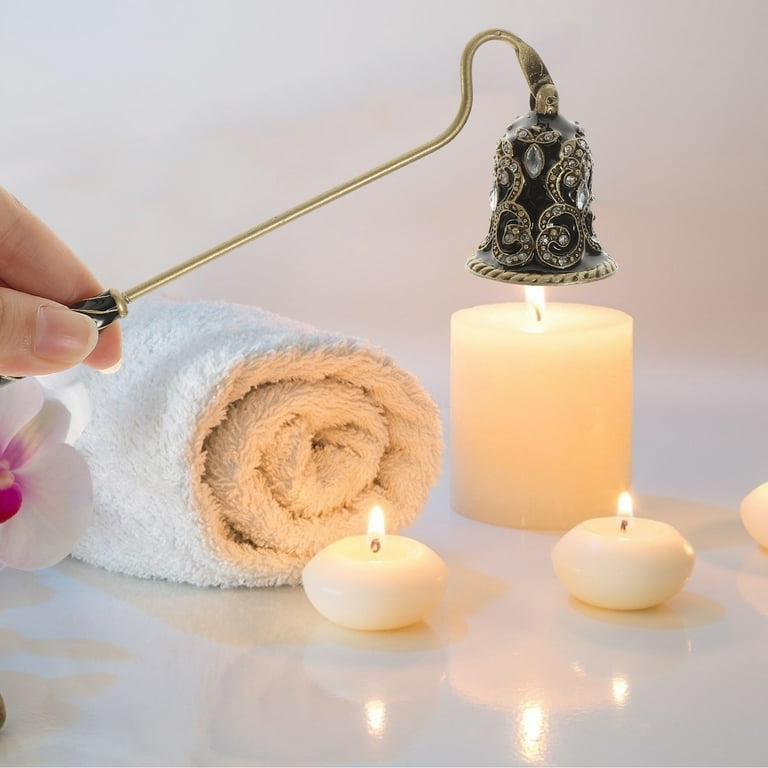The photograph captures an elegant scene with a white backdrop, featuring a small section of a hand extending from the left side, holding an ornate black and gold candle snuffer. This intricate snuffer, adorned with faux jewels and elaborate designs, is poised to extinguish a flame atop a white pillar candle. Next to this pillar candle, a neatly rolled white towel and the partial view of a pink and white orchid add to the serene setting. In the foreground, three rounded, lit candles cast gentle reflections on the shiny white surface. The soft illumination from the flames enhances the calm and sophisticated ambiance of the image.